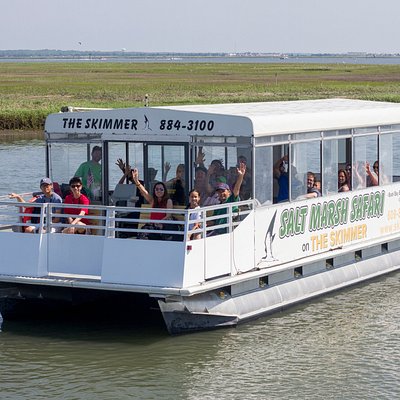The photograph captures a flatboat named "The Skimmer" on calm, pale greenish water, surrounded by a grassy, featureless field that extends to a distant horizon with blue hills. The boat is centrally positioned in the image and prominently displays the text "Salt Marsh Safari" in large green characters and "The Skimmer" in reddish characters, along with the number 884-3100. Most of the boat is roofed over with a white cover and has see-through Plexiglass windows. Passengers can be seen seated inside, looking out the windows, while a few are seated on an open deck at the front of the boat, surrounded by a fence. On this deck, one woman is waving, and others are visible, including individuals in red and blue shirts. The diverse colors in the scene include gray, blue, green, brown, white, black, yellow, and red. The setting appears to be a marshy or swamp area, contributing to the serene and scenic outdoor atmosphere.